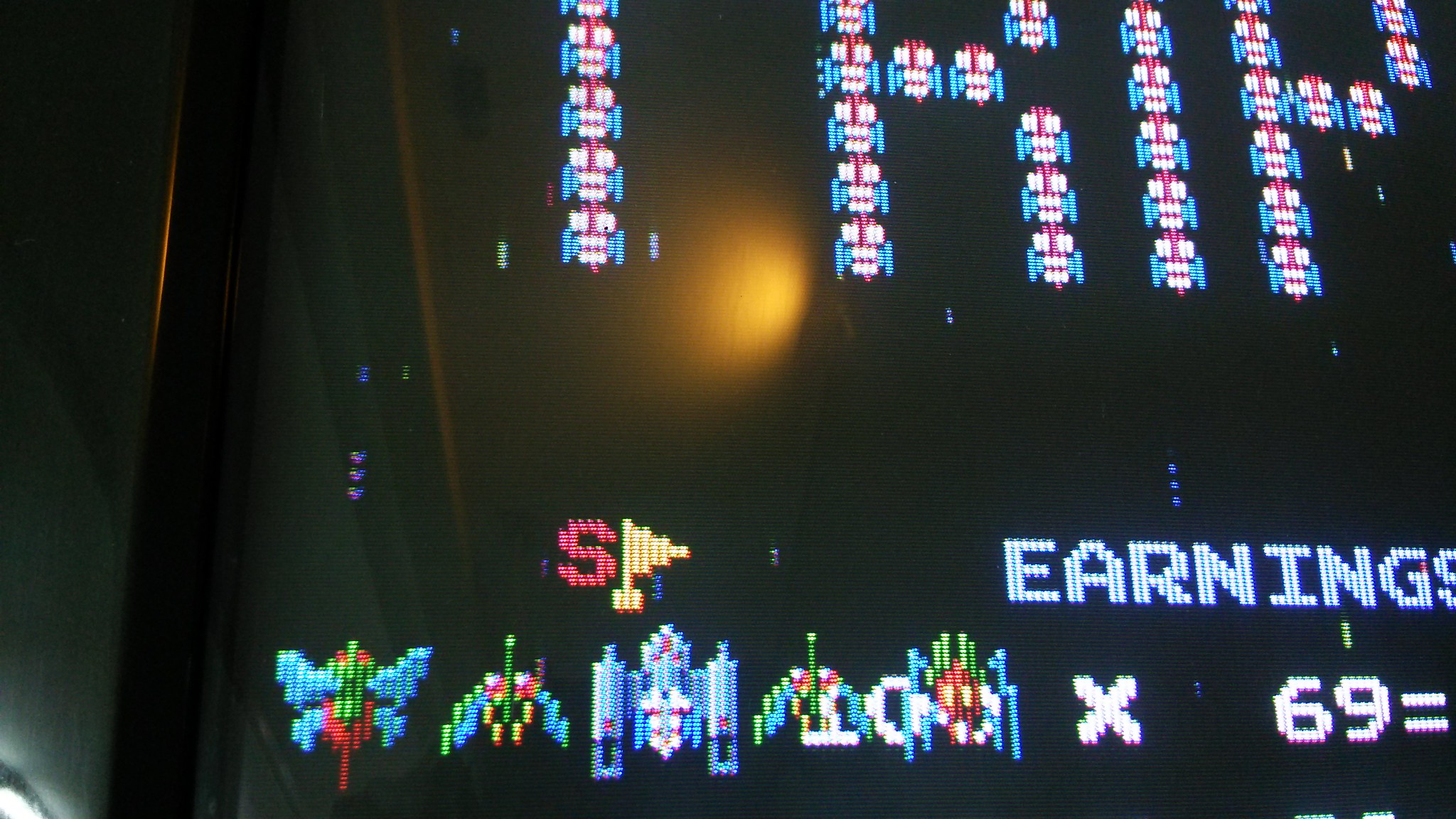The image appears to be a dark, blackish display screen about one and a half times wider than it is tall, resembling a classic CRT TV. The screen shows what looks like a results or track screen from an old-school video game, most likely Galaga. In the lower left corner, there are five horizontally arranged icons: starting with two bug-like creatures, followed by a spaceship, and then two more bug-like creatures. Up and to the right, the word "earnings" is displayed, accompanied by "time 69 =". Above this, there's a distinctive yellow flag, marked with a red "S", similar to a golf hole flag. Higher still, the screen features alien-like heads with teal wings arranged to spell out the word "TRIP", although the 'T' is lying down, almost suggesting the word "RIP". This detailed composition, iconic to classic arcade imagery, likely depicts the aftermath of a level where enemies have been defeated.